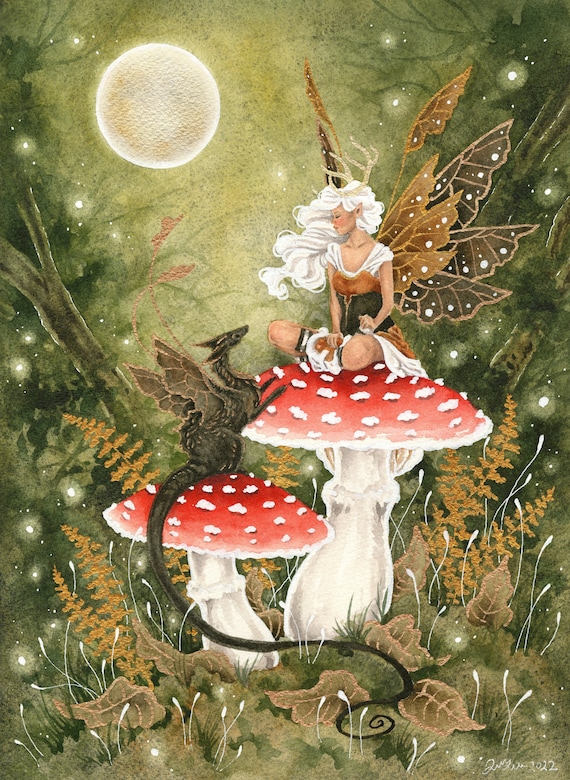In this vibrant and detailed fantasy painting, a white-haired fairy and a small green dragon are depicted in a lush, magical woodland scene filled with rich hues of tans, whites, reds, greens, and golds. Dominating the center are two prominent mushrooms with bright white stalks and vivid deep red caps adorned with white spots. The right mushroom, slightly taller, supports a fairy with dragonfly-like wings that shimmer in shades of gold and green. She sits cross-legged, wearing a white dress with a brown corset and green waist cincher, her gaze tenderly directed towards her companion. The smaller mushroom on the left is the perch for a green dragon with an elegant, long tail that curls down to the ground, wrapping around the base of the fungi. The dragon, characterized by black accents and insect-like wings, raises itself on its hind legs with the front paws resting on the right mushroom, creating a sense of interaction between the two mystical creatures. Surrounding this enchanting duo is a verdant backdrop of leafy green grasses and golden ferns, with a glowing golden moon outlined in bright white dominating the upper left corner of the canvas, casting a magical light across the scene. The ground is speckled with white lights, completing the ethereal ambiance of this fantasy landscape.